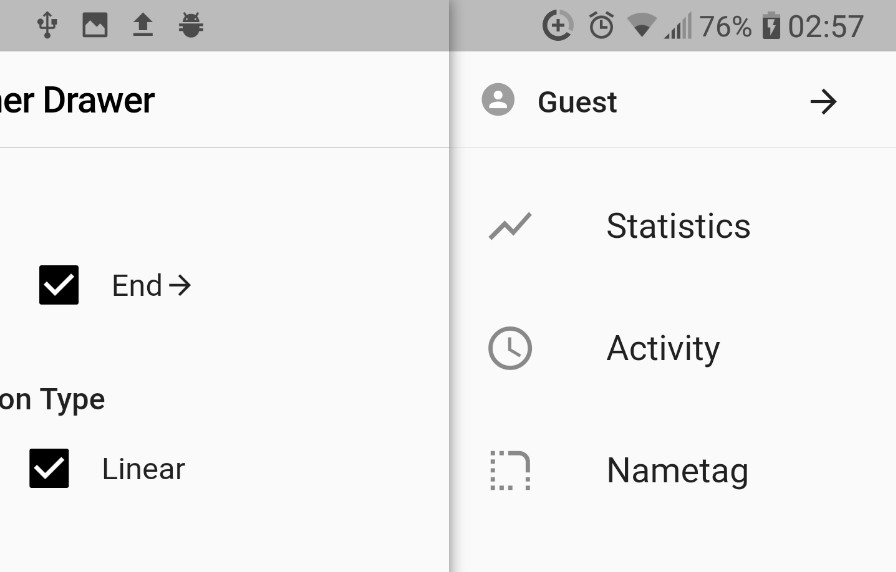This image is a screenshot of a mobile device displaying a webpage. At the top of the screen, several standard mobile icons are visible: an alarm icon indicating an active alarm, cell signal strength, Wi-Fi connectivity strength, a battery icon showing a 76% charge, and a time display reading 2:57 PM. The content of the webpage appears to be presented on a plain white background with black text and some areas of gray shading. 

There is no formal alignment or justification evident in the layout of the page's elements, which are scattered throughout the screenshot rather haphazardly. The top bar of the webpage includes information about the user's status, indicating that it is a guest account and the profile is not signed in. On the right-hand side of the screen, options are available for "Statistics," "Activity," and "Name Tag."

Checkboxes labeled "End" and "Linear" are visible, with "Linear" being selected. The simplicity of the page's design, devoid of any elaborate images or graphics apart from the essential icons and textual content, emphasizes the utilitarian function of this webpage.